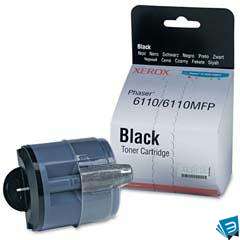This professionally taken promotional image, likely sourced from a website, showcases a Xerox black toner cartridge set against a stark white background. The focal point is the black, gray, and clear toner cartridge itself, positioned in front of its packaging. The packaging, which has a prominent white backdrop, features the Xerox logo in red at the top. Noteworthy details include the product identification number "6110-6110MFP" and the label "Black Toner Cartridge" in black text, placed prominently in the center of the box. The top of the packaging has a black strip with white text reading "black" and includes a small punched hole for hanging display, possibly for retail settings. In the bottom right corner of the image is a blue corporate logo resembling a book with a mirrored 'E' in white. Overall, the design draws attention to the toner cartridge and its packaging, similar to product listings found on major online retail sites like Amazon.